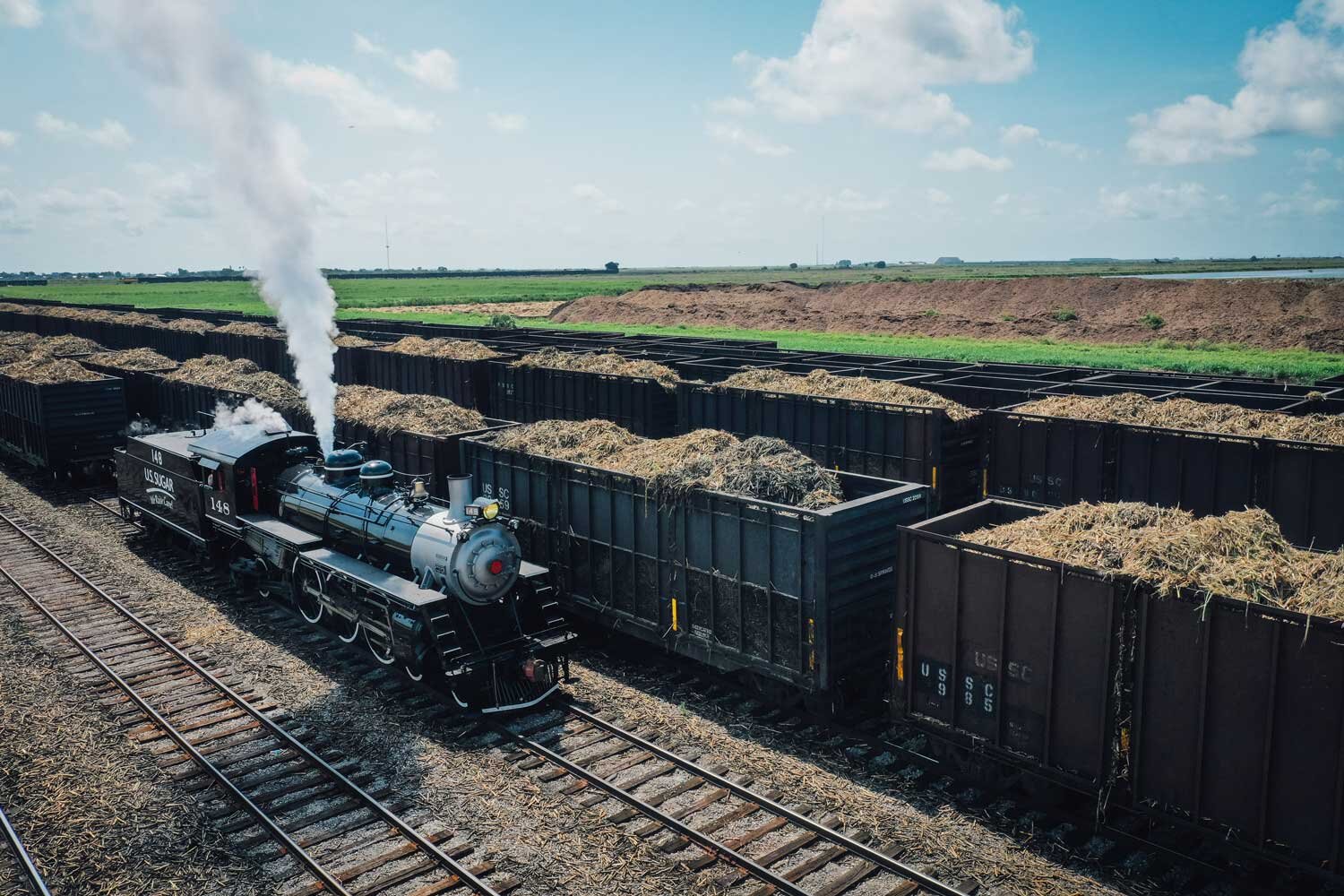This image captures a bustling train yard during the day under mostly clear blue skies with a few clouds on the horizon. Dominating the scene is a shiny and new steam engine emitting steam, seemingly ready to move. The engine is pulling a single car filled with hay, positioned on the second track from the left. To its left, there's an empty train track. Surrounding this engine are multiple rows of train tracks, housing cargo trains with open tops. The containers of these trains mostly hold hay or similar material, filling rows three through six. In the background, a vast expanse of green fields stretches out, with some houses, buildings, and possibly antennas or cell towers visible. Far off in the distance, a glimpse of a body of water can be seen, adding a serene element to the industrial scene.